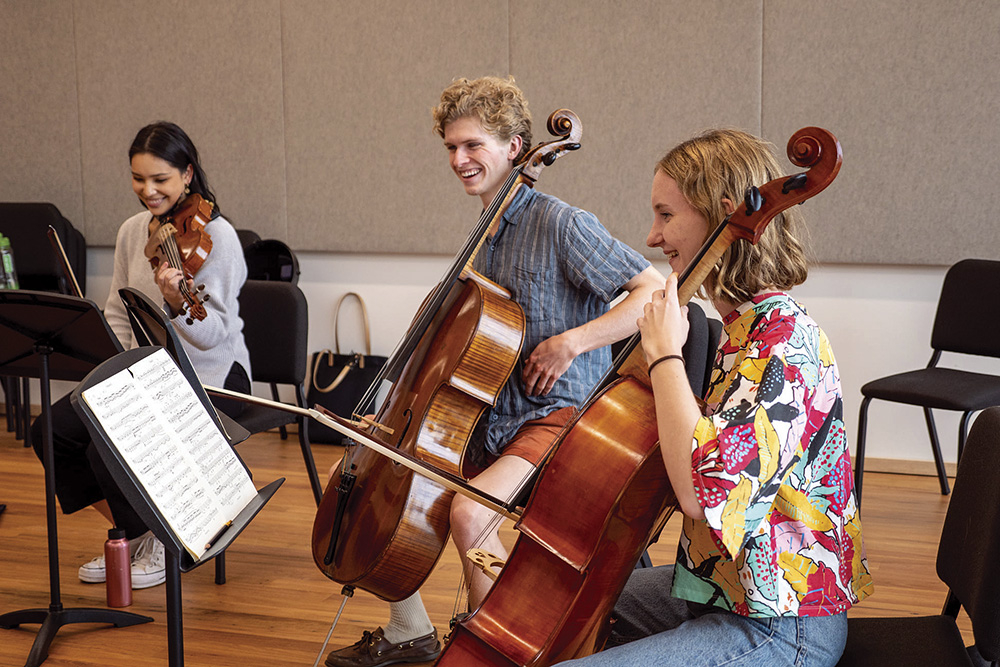Indoors, during the daytime, three young musicians are captured in a warmly lit room with golden brown wood flooring and white walls partially covered by a brown sound barrier. On the left, a young woman with long, dark hair and dressed in a gray sweatshirt, black pants, and white shoes, is playing a violin. She is smiling as she holds the bow in her right hand, looking at the sheet music on a black metal stand in front of her. In the middle, a young man with short, blonde, curly hair, wearing a blue shirt and orange shorts, is engaged with a cello. His right hand holds a bow, poised over the strings, and he, too, is focused on his music stand. To his right, another young woman, with medium-length blonde hair and wearing blue jeans and a white shirt adorned with red and yellow leaf prints, is playing a cello as well. Sitting on black chairs, all three musicians have light skin tones and are either preparing to play or currently playing their instruments, each looking at the music stand with sheet music in front of them. In the background, there are a few empty chairs and what appears to be purses, suggestive of a music practice setting.